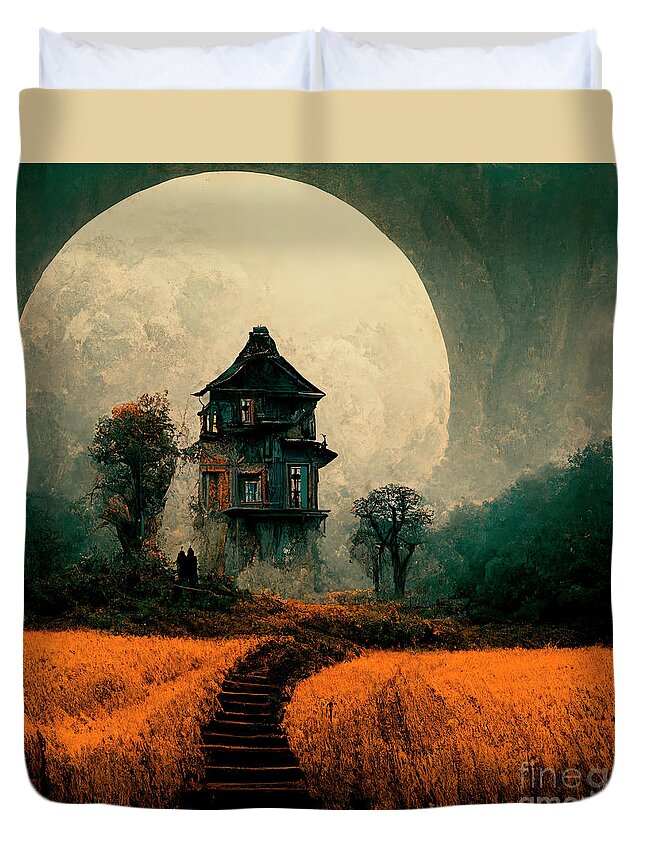This image, which appears printed on a pillowcase or digital blanket, portrays a stylized nighttime scene featuring a tall, three-story, dilapidated shack with distinctive peaked roofs. The grungy whitish-yellow moon dominates over a third of the top left corner, casting an eerie glow on the grungy green sky that fades to white at the horizon. To the left of the shack stands a large tree, while to its right is a smaller tree and a forest tree line. Below the house, a set of stairs descends into the foreground, bordered by washed-out dark yellow and black, hay-like ground or an orange field. Two shadowy figures can be seen around the house, adding to the haunting atmosphere. In the bottom right corner, the text "Finea" is visible in white lettering.